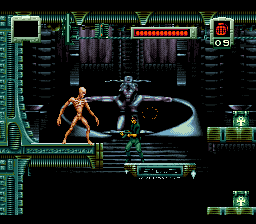In this screenshot from a video game, the main character, a small avatar dressed in a green outfit, is gripping a black assault rifle. He is positioned on a stairwell within a futuristic space station. Directly in front of him looms an imposing antagonist, resembling a humanoid skeleton and likely serving as a formidable boss in the game. Above the protagonist, the skeletal adversary appears ready to engage in battle. Adding to the scene's intensity, another character with outstretched white arms can be seen in the background, contributing to the high-stakes atmosphere of this pivotal moment in the gameplay.